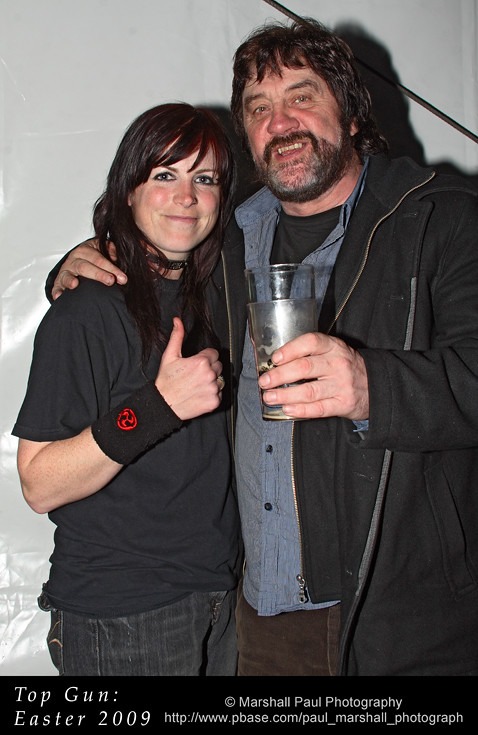In this photograph, a smiling couple stands closely with their arms around each other against a light backdrop that appears to be white or light gray. The woman, positioned on the left, has brown hair with burgundy highlights and wears a black t-shirt paired with baggy black jeans. She gives a thumbs-up with her right hand, which is adorned with a black wristband featuring a red swirl logo. Her cheeks are pink, and she wears noticeable mascara. The man has his right arm around her shoulder and holds a drink, presumably beer, in his left hand. He sports a black zip-up jacket over a gray shirt with black buttons and a black t-shirt underneath. His brown hair is slightly wavy and shows hints of graying in his beard and mustache. Both are dressed casually and exude a relaxed, happy demeanor. Below the image is a thick black horizontal line bearing the text “Top Gun: Easter 2009, Marshall Paul Photography” and a URL for the photographer’s website.